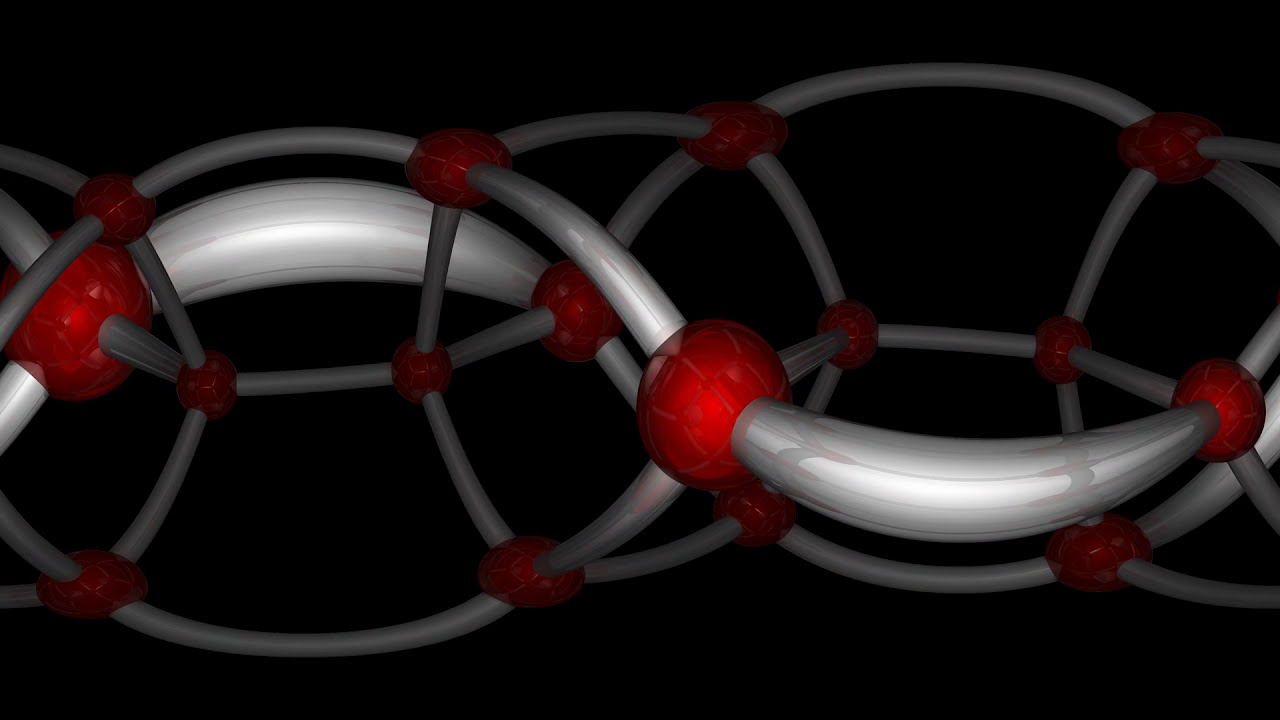The image depicts an animated, computer-generated model of a DNA helix, set against a stark black background. The DNA strand is composed of shiny silver, oblong segments that reflect light, connecting at regular intervals via red, globe-like structures resembling beads or cherries. These red circular nodes dot the entire length of the silver DNA strands, which elegantly curve from left to right and back in a smooth, undulating motion. The high-definition, widescreen format of the image further accentuates the intricate details and seamless flow of the DNA helix. The interplay of silver and red elements creates a visually striking contrast against the dark backdrop, emphasizing the dynamic and complex nature of the DNA model. The entire composition has an almost fisheye lens effect, with varying thicknesses of the cables that connect the red spheres, adding a sense of depth and dimensionality to the illustration.